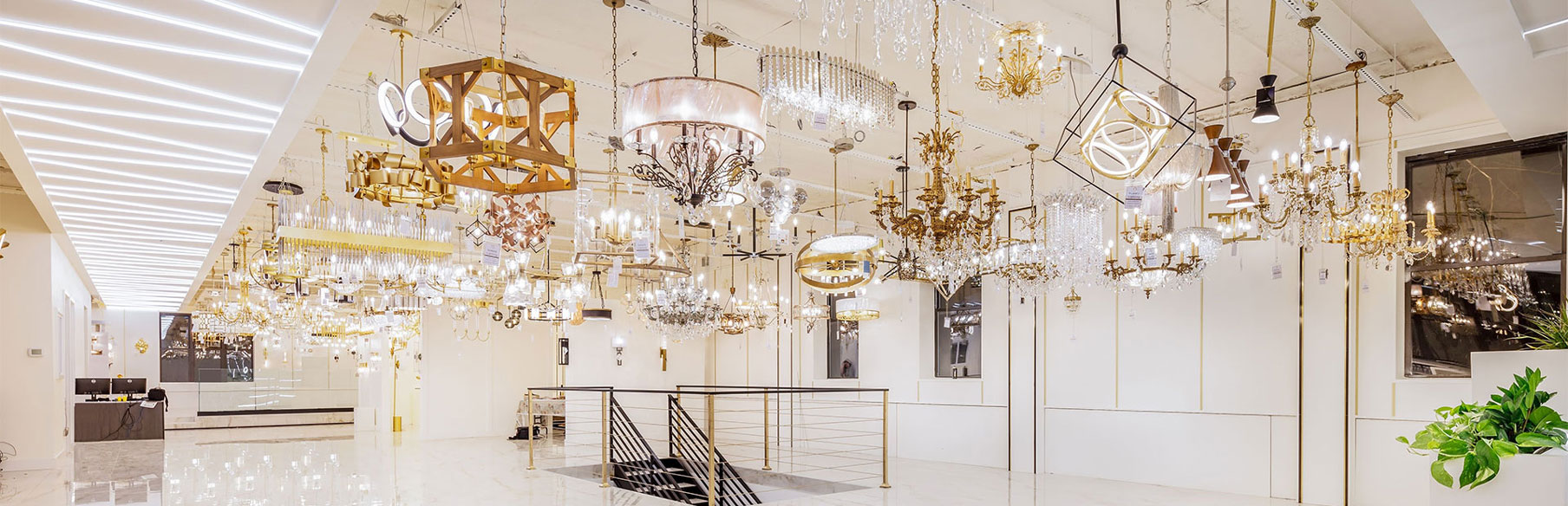This image captures a panoramic view of an upstairs room that resembles an art gallery or designer lighting showcase. Dominating the room are numerous chandeliers hanging from the ceiling, crafted in various styles and colors, including brown, gold, silver, and black, all illuminated and radiating a brilliant shine. The room features white walls adorned with faintly visible pictures, enhancing the gallery-like ambiance. On the left side, there is a band of fluorescent lighting stretching from front to back, further highlighting the decorative lighting pieces on display. Toward the back left, there are desks equipped with computers and monitors. Centrally, a staircase with black steps descends, while on the bottom right, a vibrant green plant in a vase or pot adds a touch of natural beauty. The overall layout and the intricately crafted lighting fixtures suggest a carefully curated and aesthetically striking interior space.